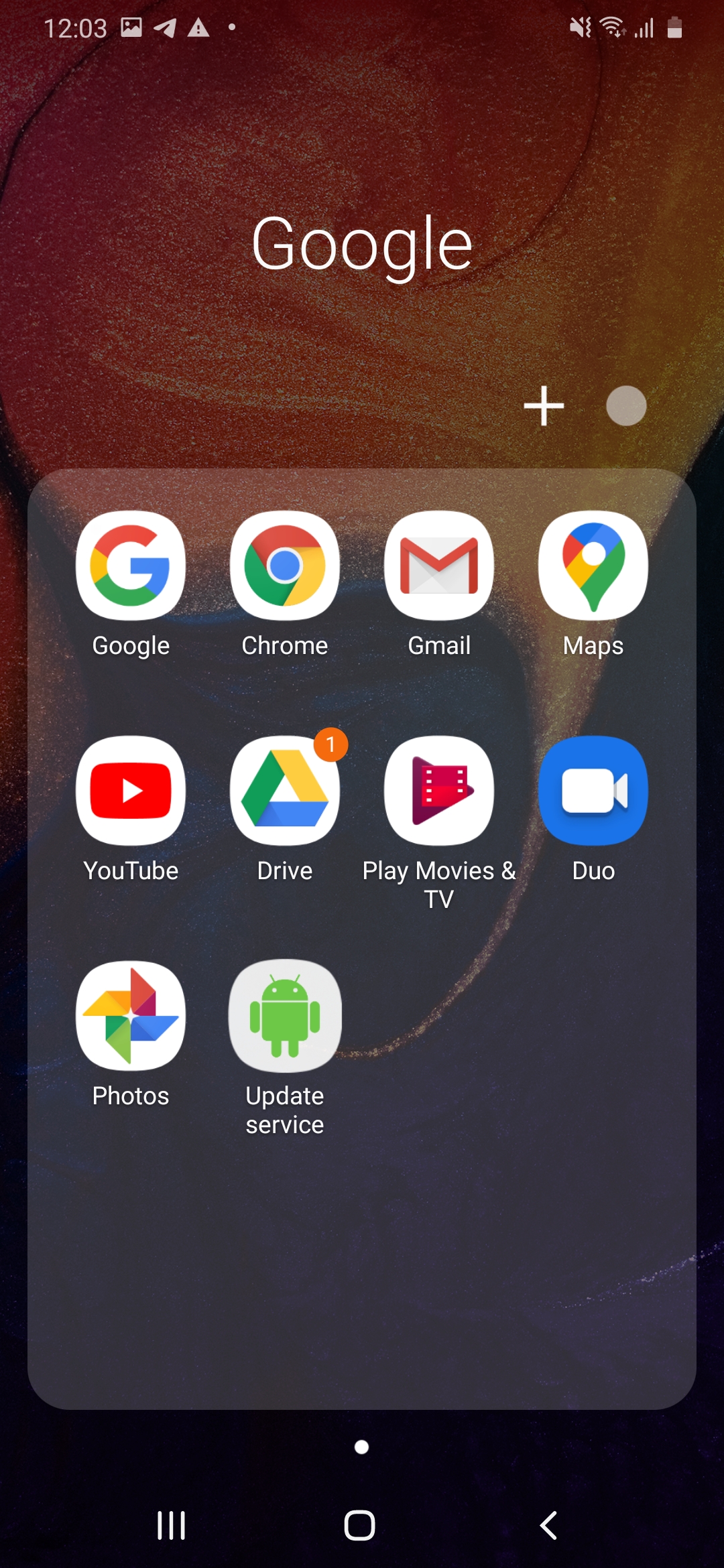The image displays a smartphone home screen with detailed elements. At the top left corner, the time is shown as 12:03. Adjacent to it are various status icons, including a caution icon depicted as a triangle with an exclamation mark, signal strength bars, Wi-Fi strength indication, and a battery icon indicating a 50% charge.

Dominating the center of the home screen is the Google search bar in white text. To its right, there is a plus sign and a gray circle. Below this, a section houses multiple app icons arranged in three rows. The top row features icons for Google, Chrome, Gmail, and Maps. The second row displays YouTube, Drive, Play Movies & TV, and Duo. The bottom row contains Photos and Update Service.

The background wallpaper is a striking design resembling a crimson red swirl, reminiscent of lava, starting prominently at the top and gradually diminishing into black towards the bottom of the screen.

At the very bottom of the home screen are three navigation buttons: on the left, an icon with three vertical lines; in the center, a square with rounded edges; and on the right, an arrow pointing to the left.